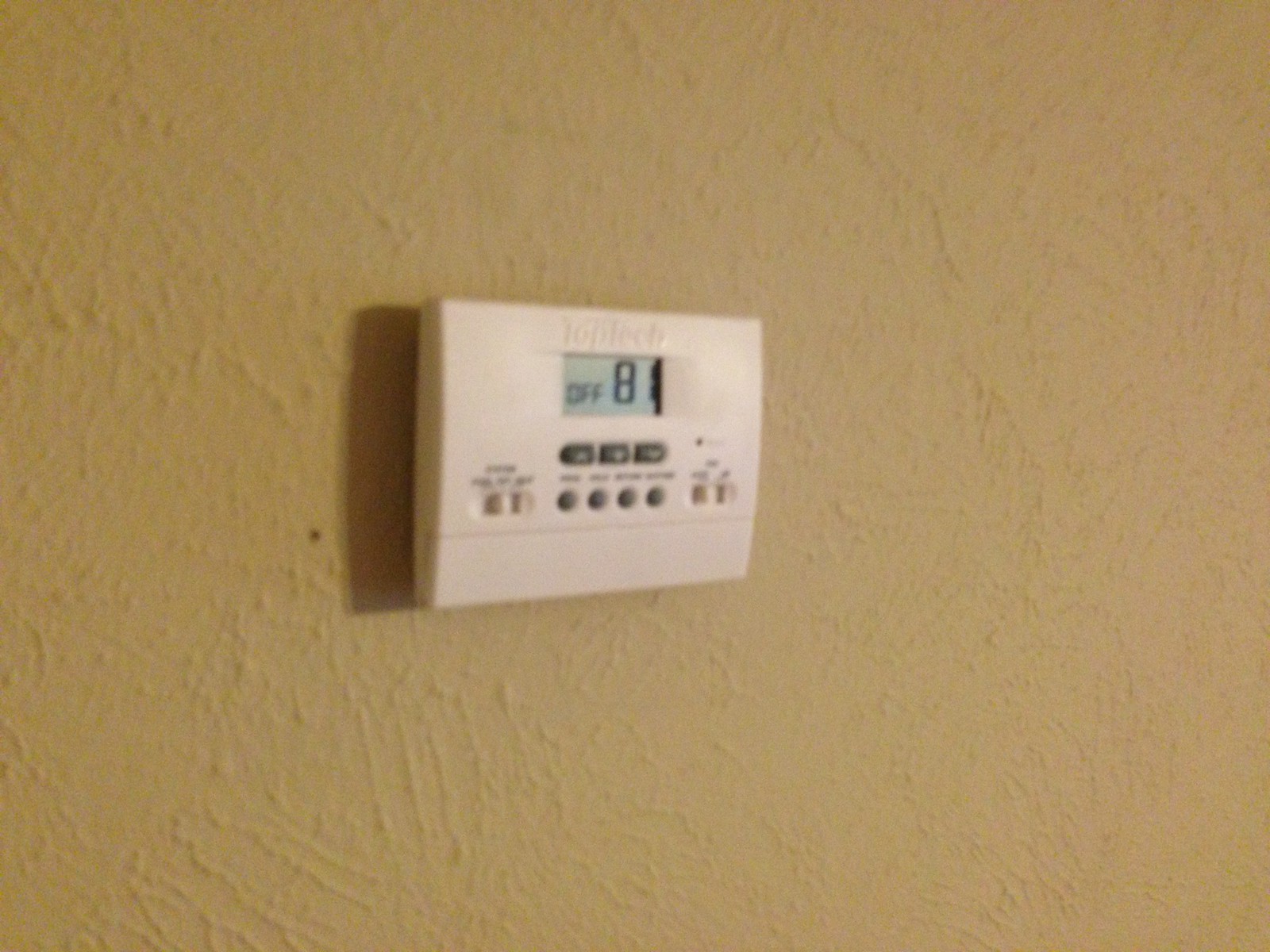In this slightly blurry photograph, we see a thermostat affixed to a highly textured wall painted in a yellowish-tan hue. The thermostat itself is crafted from cream-colored plastic and has a rectangular shape. Central to the device is a light gray display reading "OFF" with an adjacent temperature of "81." The brand name "Toptek" is subtly embossed above the display in the same color. Below the screen, the thermostat features three gray buttons, though their labels are indiscernible due to the blurriness. Further down, there are four circular gray buttons, also labeled but unreadable. On the left side of these circular buttons, a switch that can be toggled left or right is visible, yet the labeling remains unclear. Similarly, another switch is located on the right side of the four buttons, offering two selectable positions with unreadable labels.